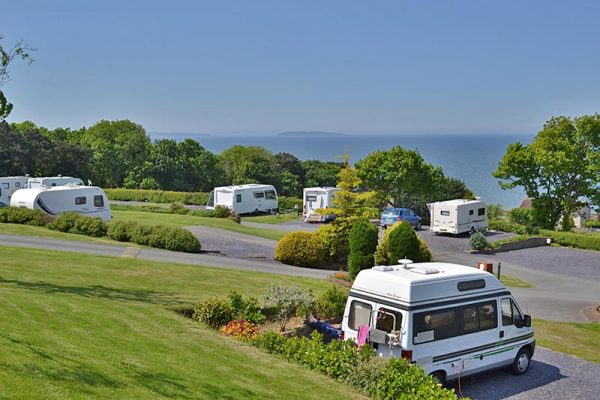This photograph captures a sunlit outdoor setting, likely a trailer park, with a distinct blue sky overhead. In the bottom right corner, a white van is parked on a concrete area, facing away from the camera and sitting near a flowerbed and some green shrubs. The van's surroundings include both concrete and dark gray asphalt. Behind the van, a winding path connects different areas, leading to a larger space populated with various white RVs, campers, and a blue minivan. These vehicles are mostly parked on an elevated, flat landscape where the grass is neatly cut, interspersed with a few bushes. In the mid-ground, a small house or building peeks out from behind a tree on the center right. The backdrop features a series of trees and hints of a body of water, possibly the ocean or a lake, with distant islands visible on the horizon.